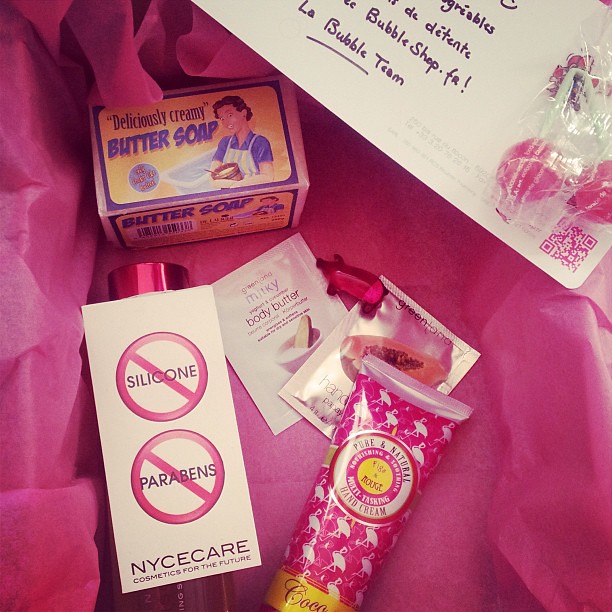The photograph depicts an assortment of household and cosmetic items neatly arranged on a pink-colored cloth, suggesting the contents of an opened gift box lined with pink wrapping paper. At the center of the arrangement is a box labeled "Deliciously Creamy Butter Soap." Accompanying this are another box emblazoned with "Nice Care Cosmetics for the Future," which prominently notes being silicone and parabens free, along with several other pink and white-themed cosmetic items. These include two small rectangular packets, one of which is identified as body butter, and another tube of hand cream described with "Pure and Natural Cream" on it, featuring a pink hue and white designs, possibly with flamingos. In the top right corner, the edge of a thank you note is visible, signed by "La Bubble Team," which is underlined, and contains a small, pink QR code. Some pink candies are also attached near the note, adding to the overall presentation.